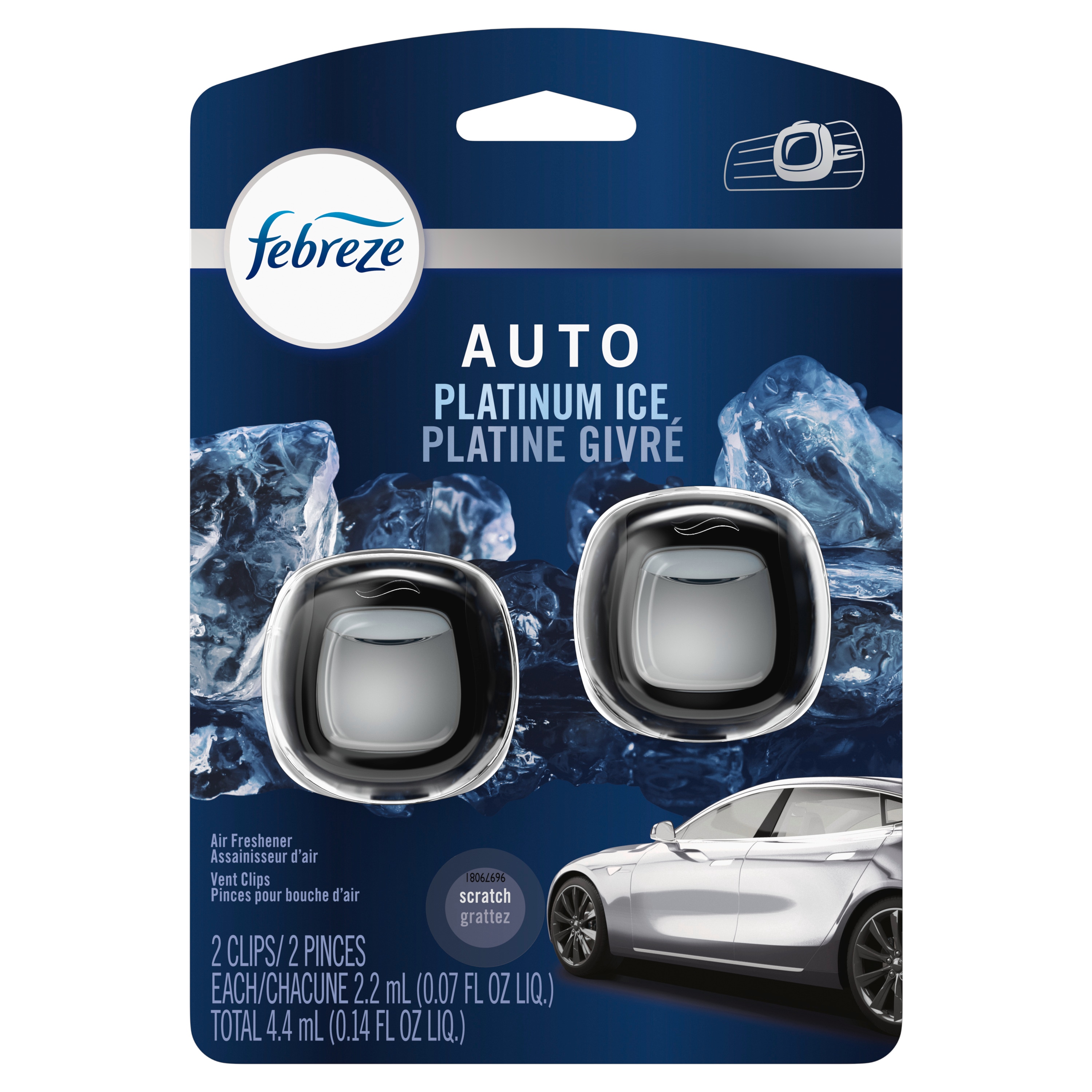The image showcases a Febreze car air freshener package set against a white background. The package is dark blue with rounded corners and a hang tab at the top for retail display. The upper left corner features the Febreze logo, a white circle with "Febreze" written in blue letters, accompanied by a small blue flourish above the word. Adjacent to this, on the upper right, is an illustration showing the air freshener clipped onto a car vent.

In the center of the packaging are the words "Auto Platinum Ice" in white and blue, followed by the French translations "Platine Givré" and “Givray”. Below this, two small, square air freshener pods are displayed—each featuring rounded corners and a central grey liquid packet. 

The lower section of the package includes instructions and descriptions: "Air Freshener" and "Vent Clips" are written in both English and French. The bottom right corner displays an image of the rear side of a silver car, while the bottom left mentions "two clips" or "deux pinces," each containing a 2.2 milliliters liquid packet, totaling 4.4 milliliters. Additionally, there's a scratch-and-sniff area labeled with English and French text. Various circle labels and numbering add detail to the packaging, enhancing its overall informative layout.